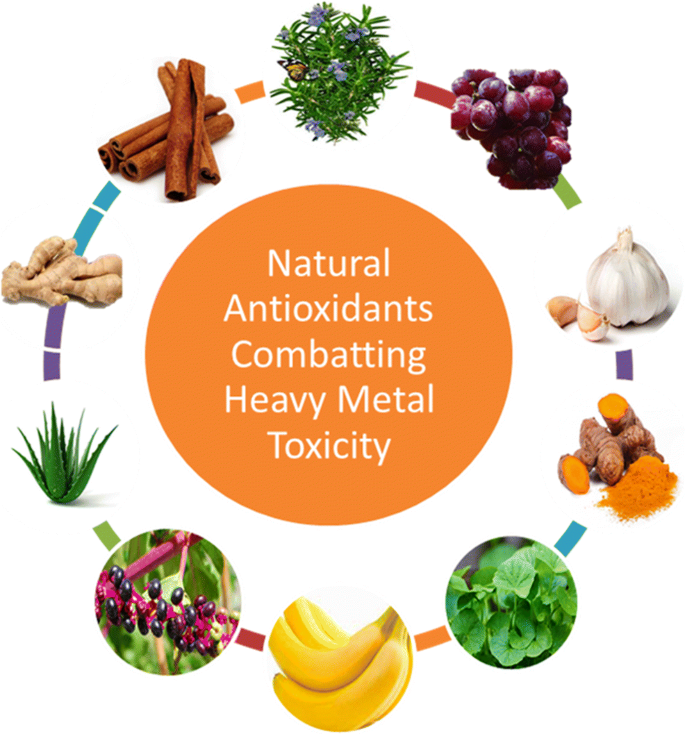This graphic features a central orange circle with the words "Natural Antioxidants Combating Heavy Metal Toxicity" written in white letters. Surrounding the circle, on a white background, are various fruits, vegetables, and herbs that exemplify the concept mentioned in the central orange circle. Starting at the top and moving in a clockwise direction:

1. At the top, there is a green herb adorned with purple flowers.
2. Next, at one o'clock, are red grapes.
3. At three o'clock, a whole garlic bulb is depicted alongside two garlic cloves.
4. Around four o'clock, there is turmeric root paired with some vibrant orange turmeric powder.
5. At five o'clock, an indistinct green leafy vegetable is shown.
6. At six o'clock, a bunch of bananas appears.
7. At seven o'clock, there are purple berries with a purple stem and green leaves.
8. At eight o'clock, an aloe plant is illustrated.
9. At nine o'clock, a ginger root is depicted.
10. Finally, at eleven o'clock, there are several cinnamon sticks.

This visual arrangement emphasizes the beneficial natural antioxidants found in these foods and their role in combating heavy metal toxicity.